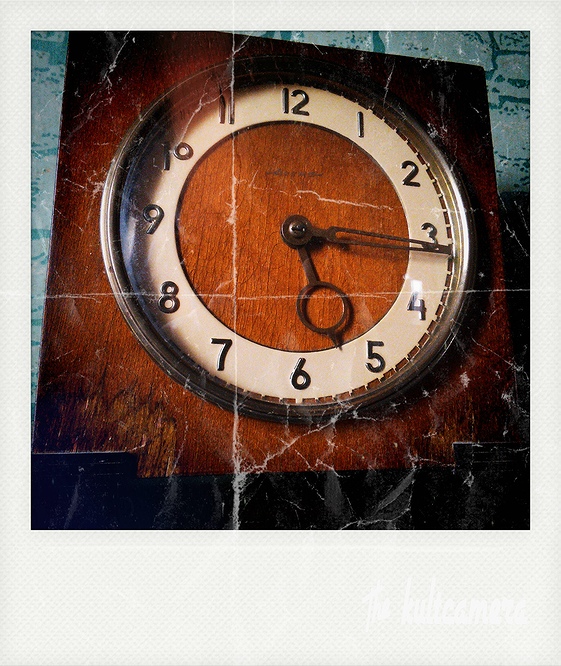This image captures an old-fashioned, distressed Polaroid photograph of a wooden mantelpiece clock. The Polaroid is framed in a white rectangle, with noticeable creases across the surface, suggesting it might be a Polaroid photo of another older photo. The clock itself, set against a weathered wooden board and a blue background, features a square dark wood frame with a round, metal-rimmed clock face. The face has numbers from 1 to 12 printed above a white ring, creating a striking contrast. The clock's hour hand features a large circle near its tip, while the minute hand is a more slender, intricate metal design. This historic timepiece provides a glimpse into the past, enhanced by the worn texture of both the clock and the photograph.